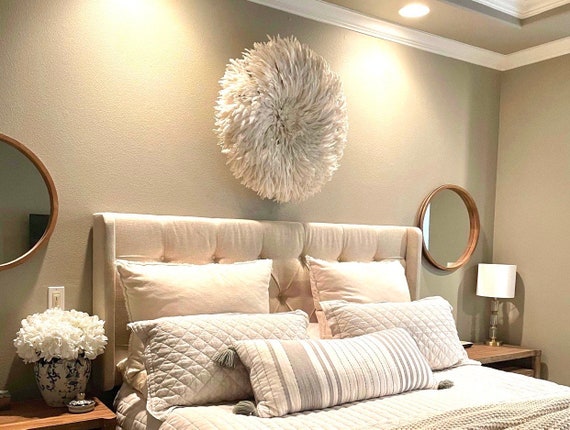The image captures a well-appointed bedroom with dark beige walls accented by white trim at the top, featuring recessed circular lights. A standout feature in the middle of the wall is a circular, feathery beige wall decoration that resembles a pillow. Below this, a bed with a light cream-colored, silky cushion-top headboard is adorned with multiple decorative pillows, including two with stitched patterns and one that is gray and cream. Flanking the bed are two wooden bedside tables, each topped with items of interest: a lamp on the right and a white-and-blue decorative vase filled with white flowers on the left. Above each table hangs a round mirror with a wooden border, reflecting the room's understated elegance.